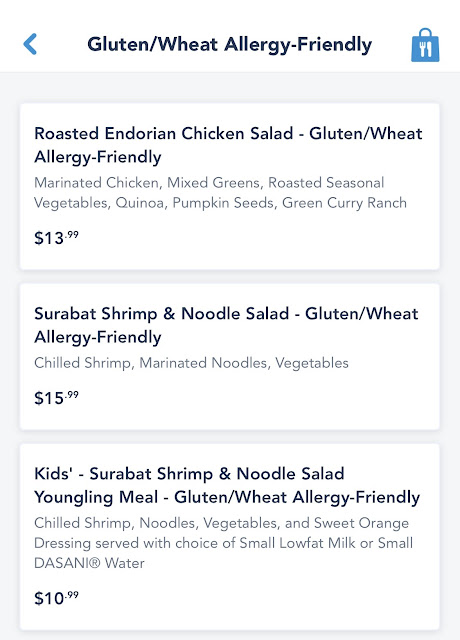Here's a clean, detailed descriptive caption based on the provided audio description:

---

Screenshot from a food website:

The image has a white background with a blue arrow pointing to the left. Centrally located black text reads "Gluten/Wheat Allergy-Friendly." Below the text is an image of a blue shopping bag featuring a white fork and knife on it.

On a gray background, there are three green boxes, each containing black and gray text detailing food items:

1. **Roasted Enduron Chicken Salad / Gluten-Free, Wheat Allergy-Free** 
   - Gray text: Marinated chicken, mixed greens, rotisserie, seasonal vegetables, kootu, pumpkin seeds, curry, green curry ranch. 
   - Black text: $13.99.

2. **Cervix Shrimp and Noodle Salad / Gluten/Wheat Allergy Friendly** 
   - Gray text: Chill shrimp, marinated noodles, vegetables.
   - Black text: $15.99.

3. **Kids' Sorbet Shrimp Noodle and Salad Younglings Meal / Gluten/Wheat Allergy Friendly** 
   - Gray text: Chill shrimp, noodles, vegetables, sweet orange dressing, served with a choice of small low-fat milk or small Dasani water.
   - Black text: $10.99.

---

Thank you to Matt and the team, as they seem to be wrapping up today.